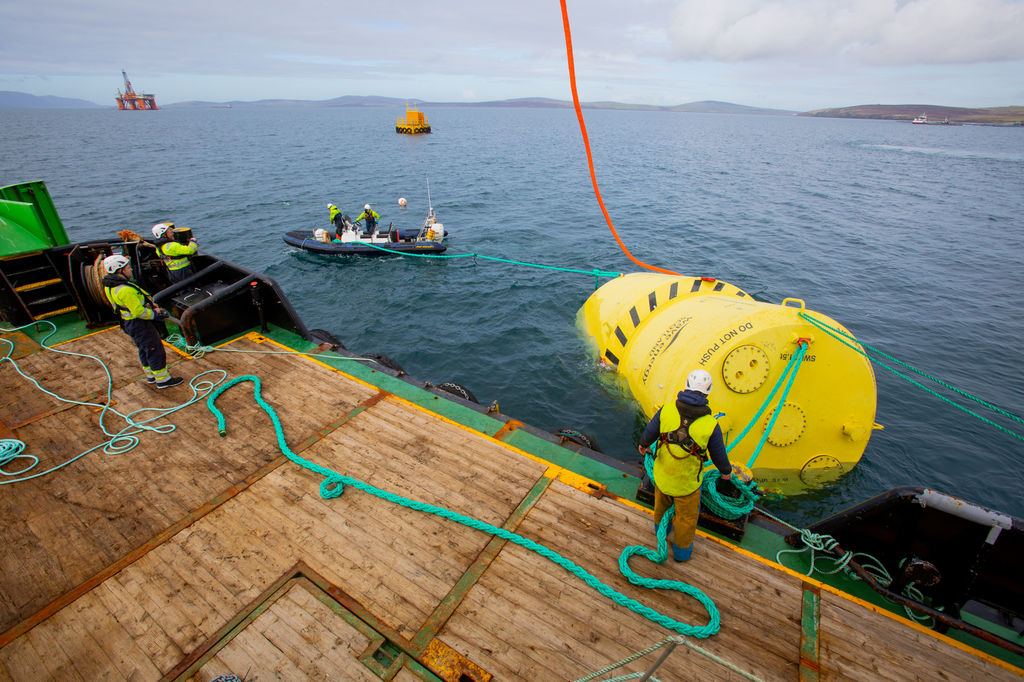This photographic image captures an outdoor scene during the daytime featuring a group of men working on a wooden dock near a body of blue-green water. The dock, adorned with a green chain running along its edge, hosts several men dressed in black clothing, fluorescent green safety vests, and white helmets. In the top left corner of the dock, two men are standing, while another man can be seen in the bottom right section, separated by the floating green chain attached to a bright yellow cylindrical structure in the water. This cylinder, marked with red and gray ropes as well as the inscription "Do Not Push" and something related to energy, appears to be a significant piece of equipment, possibly the size of a pickup truck. Nearby, two workers stand in a light inflatable raft, assisting with the equipment handling. In the background, a red oil rig floats on the upper left horizon, and a smaller floating building is visible in the middle of the image. The scene is set against a backdrop of gentle rolling hills and a light blue sky filled with grey clouds, indicating a somewhat cloudy yet bright day.